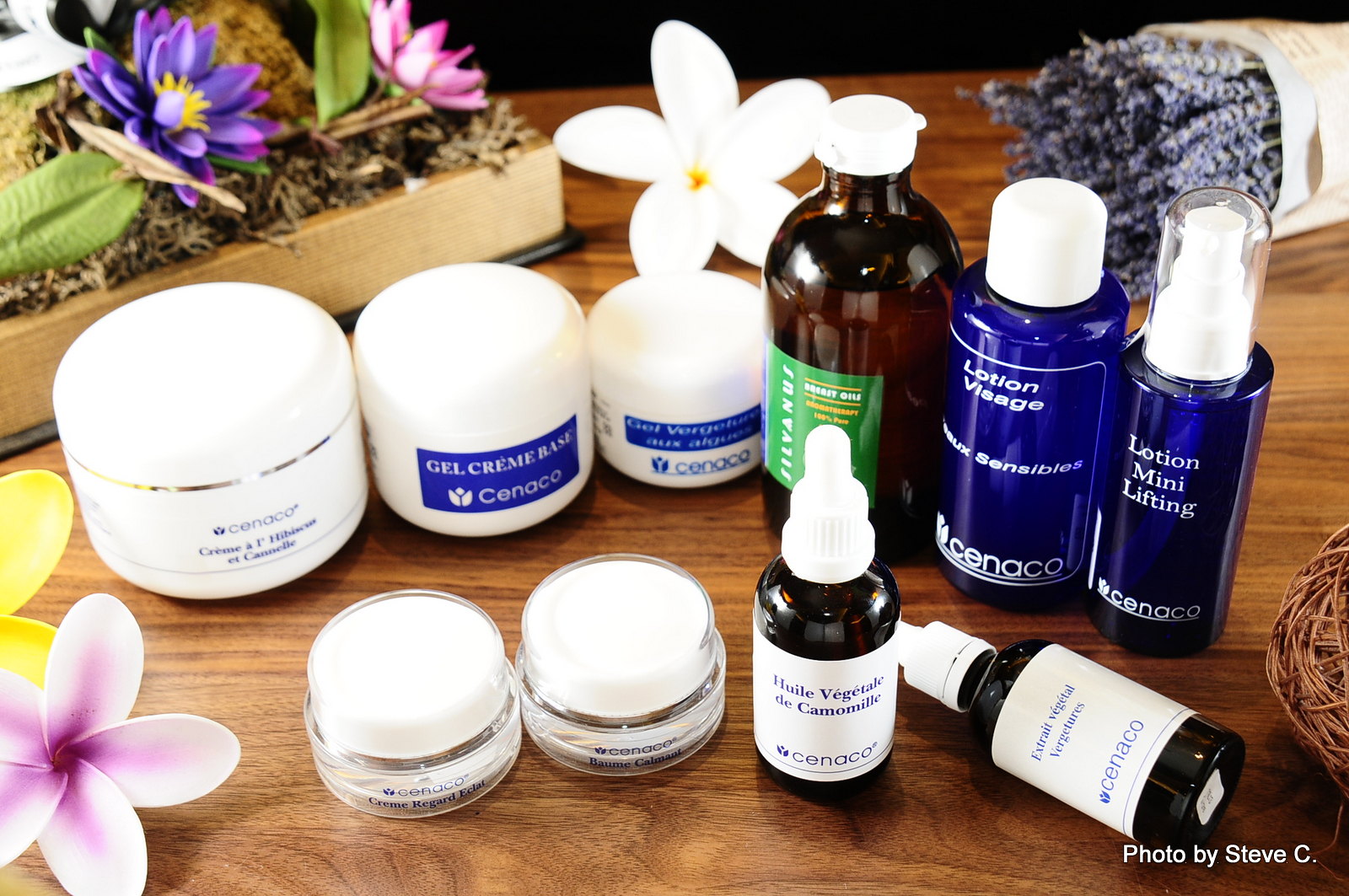The image depicts a collection of various beauty products and lotions arranged on a wooden table. In the top left corner of the table, there is an elegant display featuring a rectangular, angled box filled with potpourri and a mix of vibrant flowers. This display includes purple flowers with yellow centers, pink blossoms, and green leaves attached to brown stems. Additionally, in the bottom left-hand corner, two distinct flowers with pink centers and white outer petals can be seen next to some yellow petals.

In the foreground, positioned towards the bottom right, there is text stating "photo by Steve C." in white font. The main focus includes two small, cylindrical cream bottles with the "Cenaco" (C-E-N-A-C-O) logo. These are either plastic or glass bottles with white, circular caps. Alongside, there is a dropper bottle featuring a chamomile product, and another product marked with "extra something" also from Cenaco, lying on its side with a white label and blue fonts.

Behind this front row, there are six additional products. On the far right, two blue plastic lotion bottles with white caps are seen, next to a brown bottle with a white cap, which has a green-themed label with yellow and white elements. The remaining three products in this row are different-sized bottles from Cenaco - large, medium, and small, showcasing labels that mention gel cream, another type of cream, and a vegetable-based product. These bottles are predominantly white, maintaining a cohesive and organized display of beauty products.